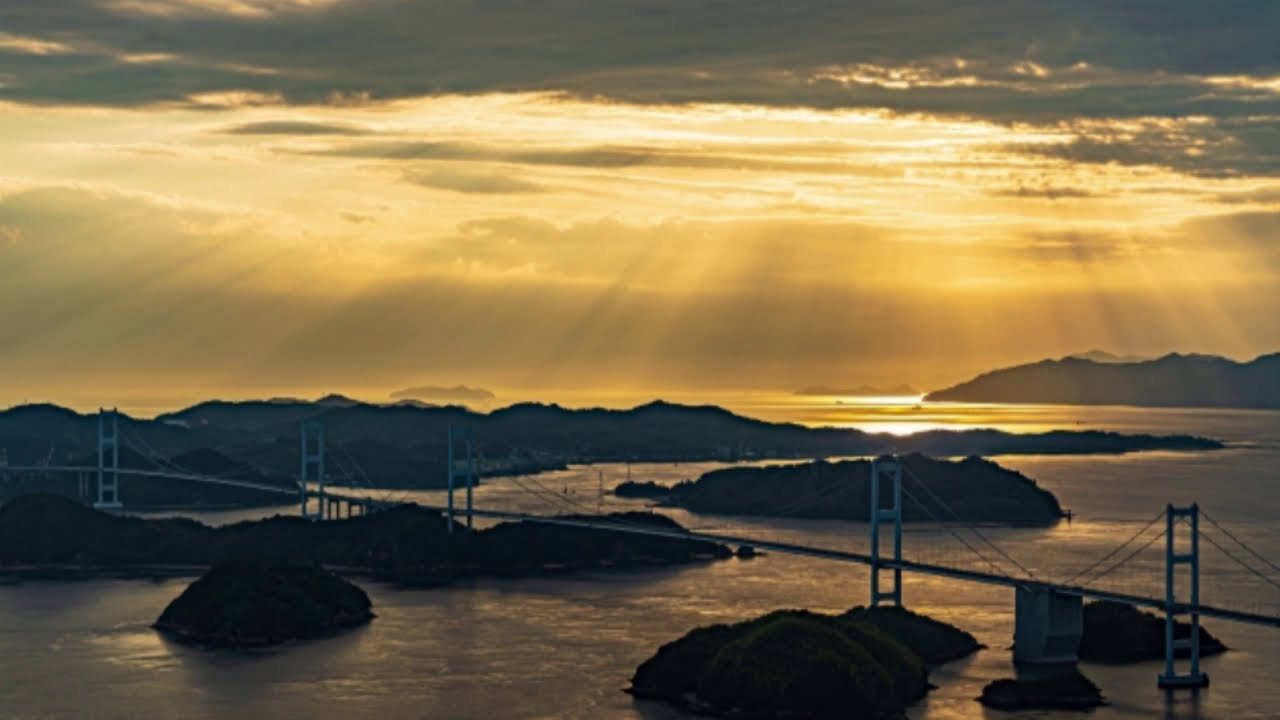The image captures a picturesque sunrise or sunset over an expansive bay with a large body of water in the foreground. The scene is dominated by a long, silver bridge with five support structures, elegantly stretching from about a third of the way up on the left side to near the bottom on the right edge of the image. The water, tranquil and vast, spans the lower half of the image, dotted with small, potentially man-made islands and patches of land adorned with trees and vegetation. The sky, which occupies the upper half, is partly cloudy with the sun hidden behind the clouds in the upper right, casting golden rays in a triangular pattern that illuminate the scene in shades of gray, golden yellow, white, and hints of brown. Notably, there are no cars on the bridge, no boats on the water, and no planes in the sky, adding to the serene and undisturbed nature of the landscape. The field of view suggests an area that spans two to three hundred feet wide, capturing a peaceful, natural setting at the edge of the day.